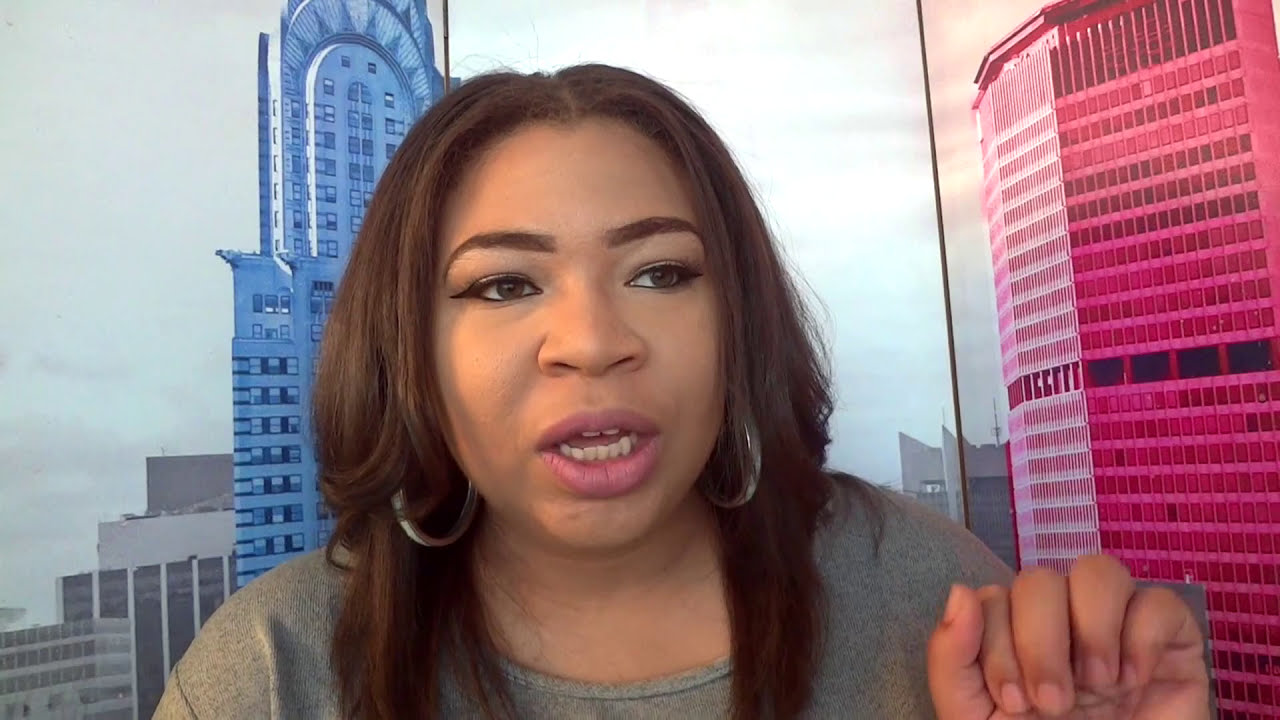In this image, a Latina woman with large hoop earrings and brown hair, dressed in a gray shirt, is centered in the frame. She appears somewhat distracted, gazing slightly off to the side, with her hand clenched in a fist. Her expression shows her teeth and red lips, suggesting a direct and focused demeanor. Behind her is a painted or printed backdrop featuring a mix of buildings in red and blue, set against a gray sky. The photograph uses a palette of light and dark blues, various shades of gray, black, brown, pink, purple, and tan. The setting seems to be indoors, possibly within a recording studio, with no visible text in the image.